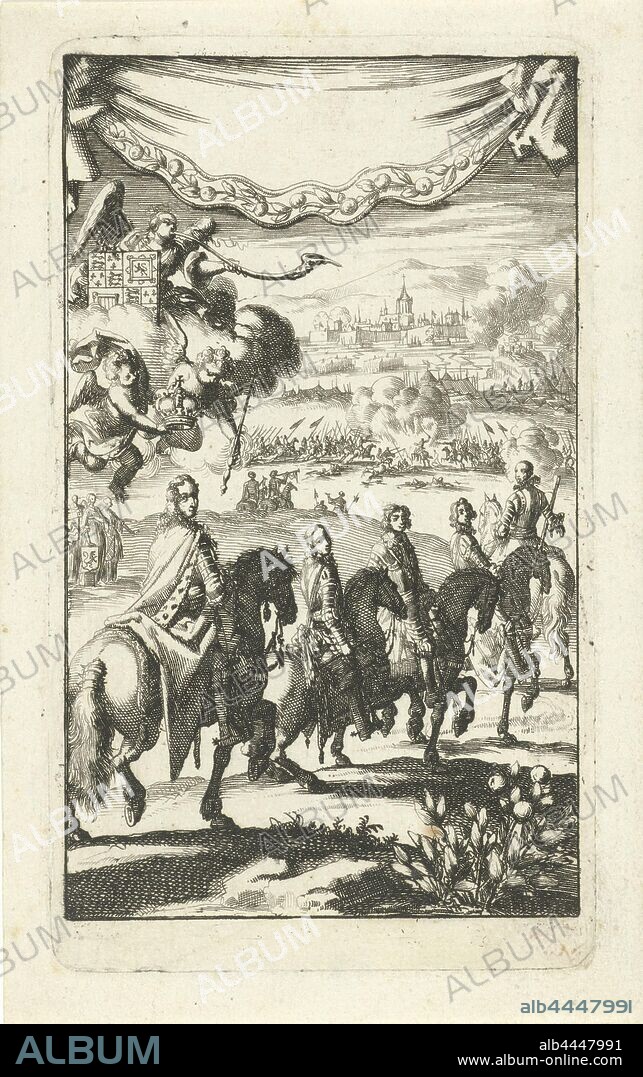This is a detailed black-and-white pen drawing depicting an intense battle scene, reminiscent of historical clashes from centuries past. In the foreground, there is a dense flower bush growing near the bottom right corner. Above it, five armored men on horseback, draped in capes, are seen riding away from the viewer, yet looking back over their shoulders, adding a sense of urgency and tension. Their outfits, reminiscent of war attire, underline the imminent conflict. Behind this group, the middle ground reveals a chaotic battlefield, rife with soldiers wielding flags and spears, engulfed in smoke and explosions. The distant city appears ablaze, contributing to the overall atmosphere of destruction and conflict. At the top left, winged angels and cherubs hover among the clouds, observing the turmoil below, while a dramatic tapestry-like banner stretches across the upper portion of the image, adding a divine or fateful aspect to the scene. This evocative drawing, marked by intricate details and emotional intensity, captures the vivid clashing of past civilizations.